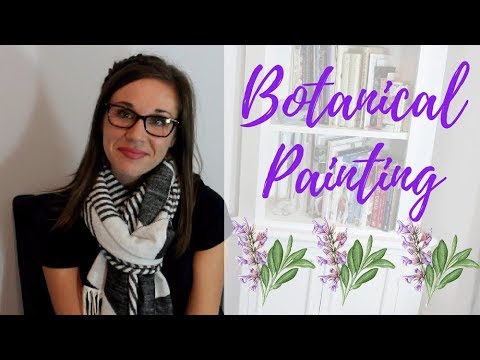This image features a white woman with medium to long straight brown hair, parted on the side with bangs, suggesting a half-up, half-down style. Her hair cascades around her shoulders as she sits in a black chair against a white wall. She wears black-framed glasses and a simple black t-shirt. Tied around her neck in a knot is a large black-and-white patterned scarf, which adds a touch of elegance to her outfit. The woman has a subtle yet cheerful smile. Overlaid on the right side of the image is semi-translucent purple text that reads "Botanical Painting." Directly below the text is a depiction of a flower with leaves, repeated three times. Behind this overlay is a tightly packed small white bookshelf, filled with books. This image appears to serve as a thumbnail for a YouTube video about botanical painting.